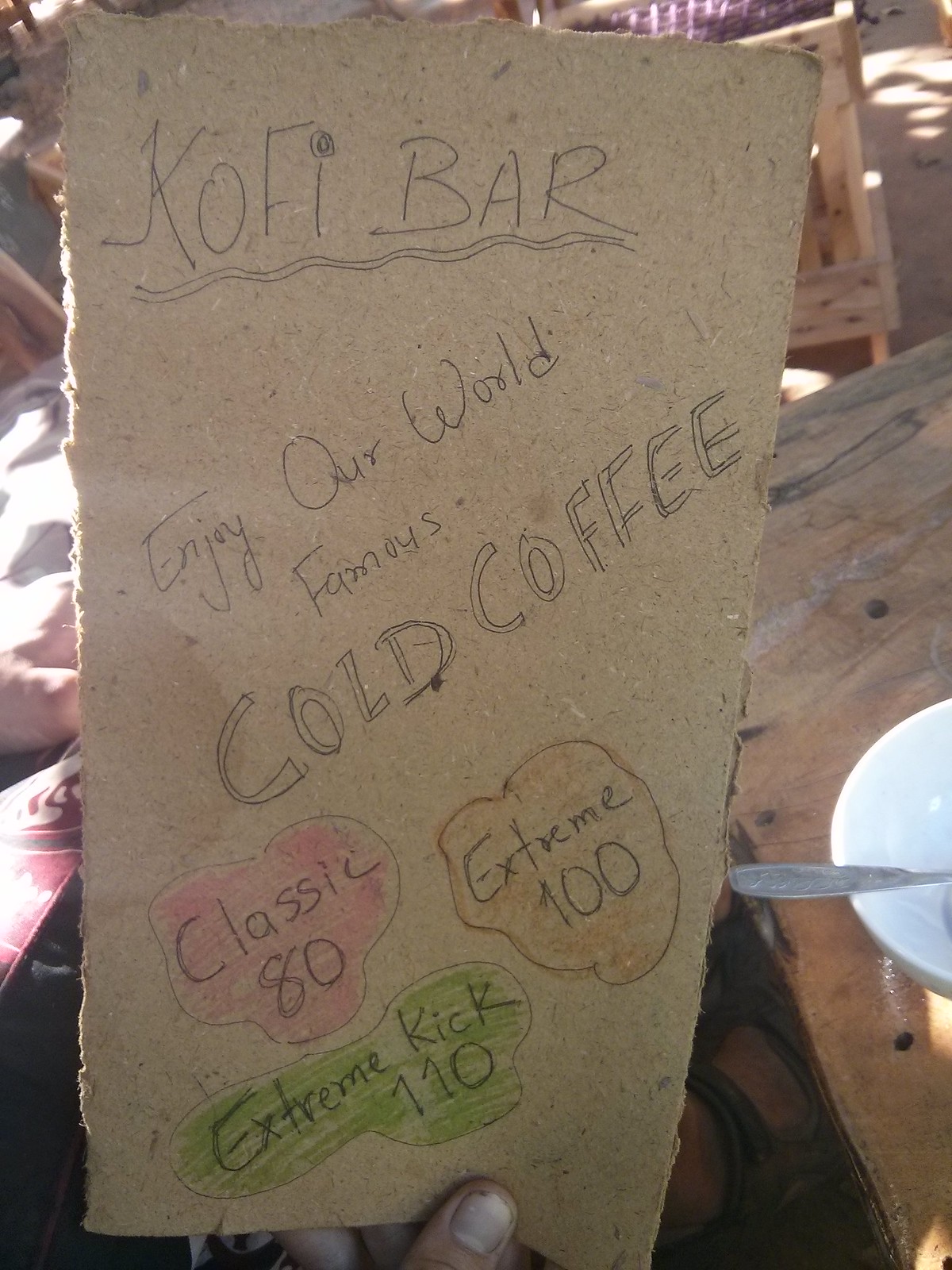This image depicts a hand-drawn advertisement on a piece of brown cardboard, held by a person whose thumb is visible at the bottom. The sign is crafted using a ballpoint pen and features a variety of embellishments. At the top, "Kofi Bar" is written in bold letters and double-underlined with squiggly lines for emphasis. Diagonally beneath this, the slogan "Enjoy Our World Famous Cold Coffee" is written in a cursive-like, stylized font, with "Cold Coffee" prominently bolded to stand out. Below the slogan, the sign showcases three irregularly-shaped word bubbles filled with crayon: a pink one labeled "Classic 80," an orange one labeled "Extreme 100," and a light green one labeled "Extreme Kick 110." This charming, homemade sign appears to be a menu or advertisement, likely for a roadside coffee stand, and captures a quaint, artisanal feel.